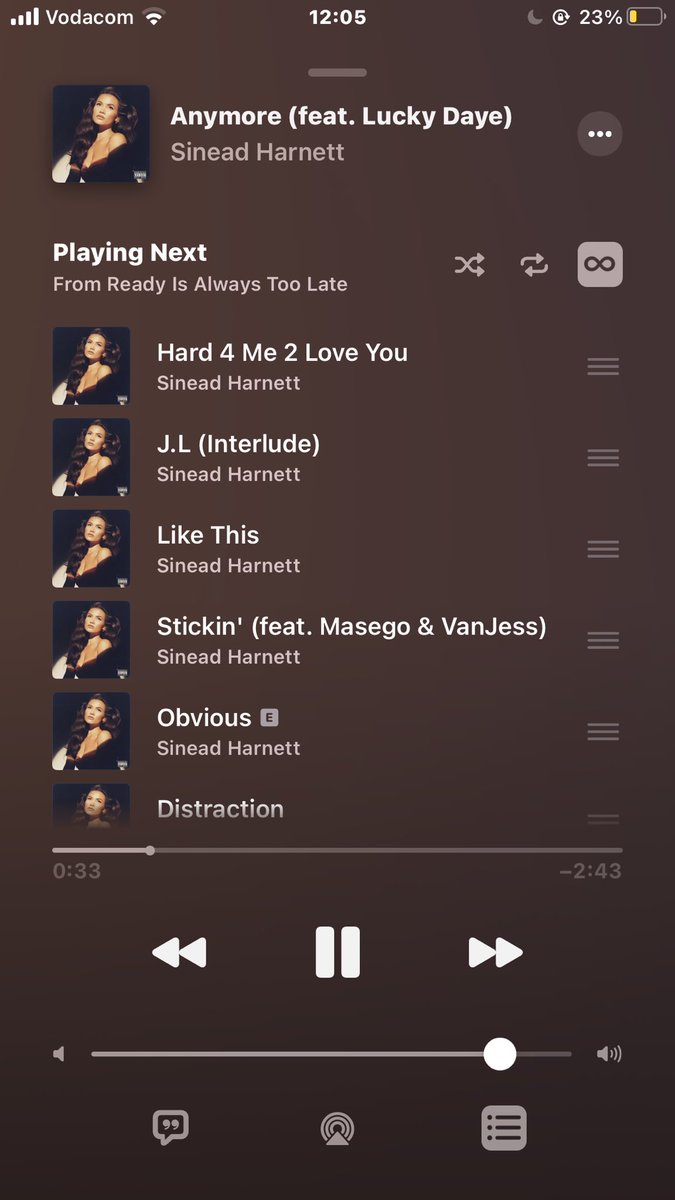This image, evidently taken on an iPhone, provides a detailed glimpse into the user's current phone activity and settings. The screen shows that the user is subscribed to Vodacom as their cellular provider and is connected to Wi-Fi. The time displayed is 12:05, and the phone has both the "Do Not Disturb" mode and screen orientation lock activated, ensuring that the display remains in portrait mode regardless of how the phone is tilted. The battery is at 23%, but the user has enabled Low Power Mode to prolong battery life.

The foreground of the image focuses on the Apple Music interface, where the user is currently listening to "Anymore" by Sinead Harnett, featuring Lucky Daye. The song is 33 seconds into its 2-minute and 43-second duration. The upcoming queue features several more tracks from Sinead Harnett's album, including "It's Hard for Me to Love You," "JL, The Interlude," "Like This," "Stickin" featuring Masego and VanJess, "Obvious" (marked as explicit), and "Distraction."

Additionally, the current setup allows the user flexibility in managing their music queue, with options available to reorder the upcoming tracks as desired.